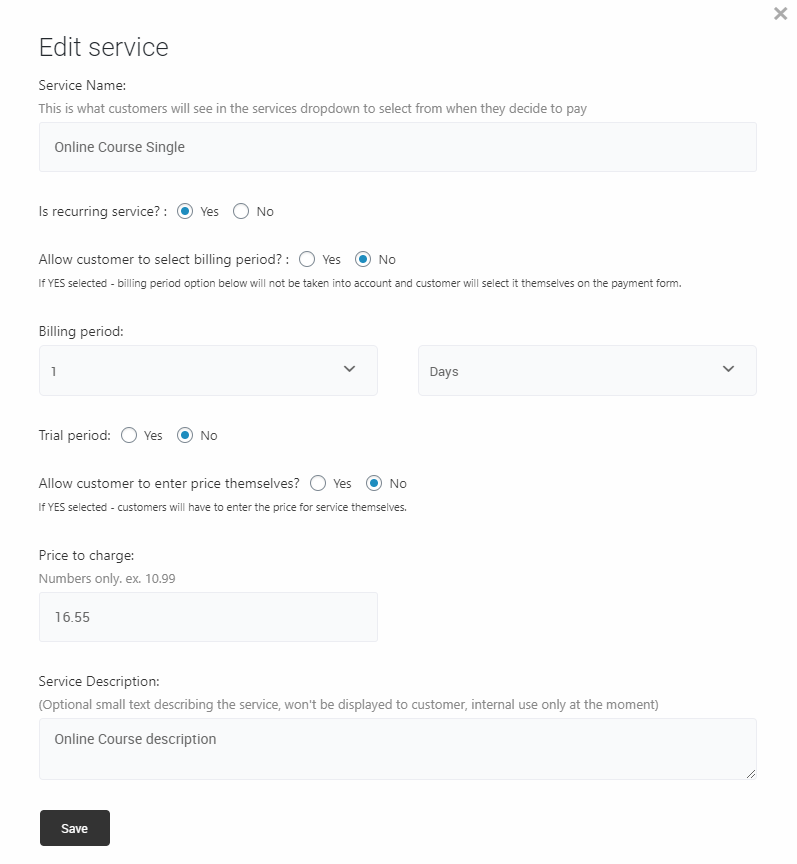Screenshot of a Payment Configuration Web Page:

The screenshot captures a web page interface designed for configuring payment services. The page sports a clean, minimalistic look with a predominantly white background. At the top of the page, in bold black lettering, the heading reads "Edit Service: Service Name". This section explains that this is the name customers will see in the drop-down menu when selecting a service to pay for.

Beneath this heading, there is an input box labeled "Online Course Single". Following this, a section labeled "Is Recurring Service" is displayed with two radio buttons for selecting "Yes" or "No". The "Yes" option is selected, indicated by a blue circle.

Next, there's a prompt stating "Allow customer to select billing period," accompanied by another set of "Yes" and "No" radio buttons, with "No" currently selected. An explanatory note below clarifies that if "Yes" is selected, customers will choose their billing period on the payment form and the default option below will not apply.

Immediately below, there are options for setting the billing period, featuring a dropdown menu with the option "1", and another dropdown menu beside it labeled "days."

Following this are options for "Trial Period," again with "Yes" and "No" radio buttons; the "No" option is currently active.

The next section addresses whether customers can enter the price themselves. The "Allow customer to enter price themselves" option also has "Yes" and "No" radio buttons, with "No" selected. An accompanying note indicates that if "Yes" were chosen, customers would have to input the service price themselves.

Further down, there's a field labeled "Price to Charge" for entering the price in numbers only, with an example given (e.g., 1099), currently filled in with "$16.55".

Towards the bottom, there's an optional "Service Description" field for internal use. This field states that it is not visible to customers and is currently filled in with "Online Course Description".

The page concludes with a black button featuring white text that reads "Save," ready to finalize any configuration changes made by the user.

Overall, the page is structured to ensure clear and precise configuration of payment options, providing both drop-down menus and radio buttons for a user-friendly experience.